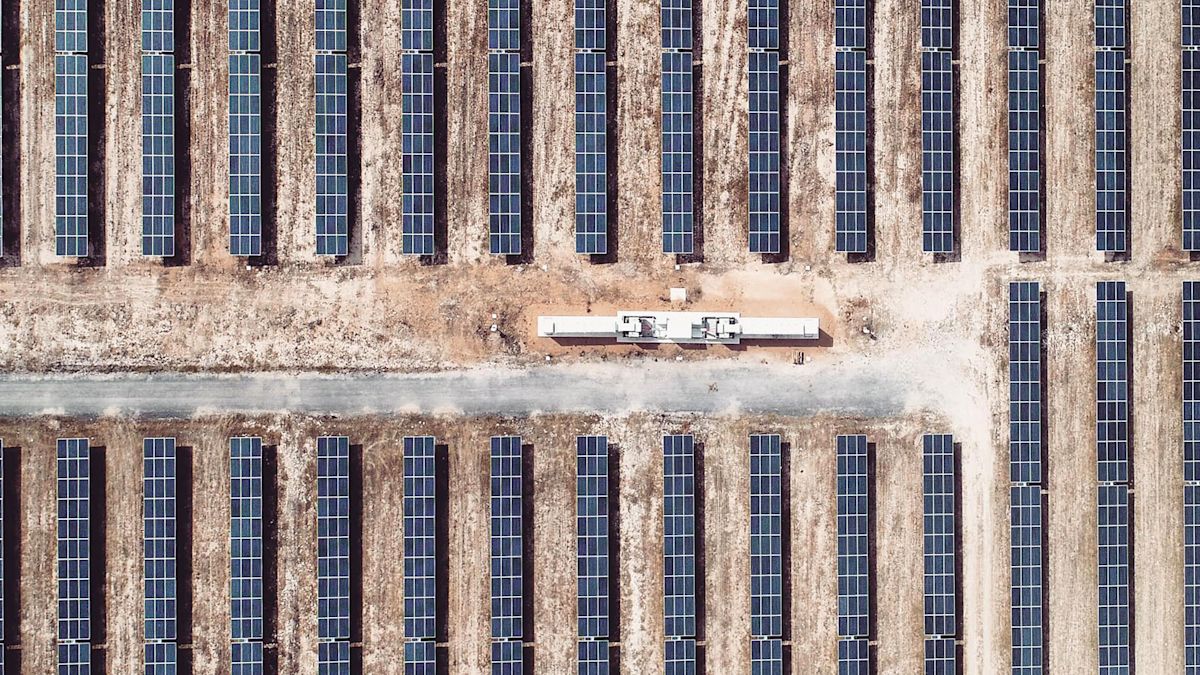This aerial photograph showcases a vast solar panel farm consisting of multiple neatly arranged rows of solar panels, positioned in a dirt field. The panels, characterized by their reflective shades of purple and blue, are organized into approximately 10 to 12 rows, with notable consistency across each row—each hosting around fourteen individual panels. Centrally located within the array is a significant white building, possibly serving as the operational hub for the farm, with additional white container-like objects scattered nearby. The clean and symmetrical arrangement of the solar panels, combined with the central structures, highlights the organized and functional design of this renewable energy installation.